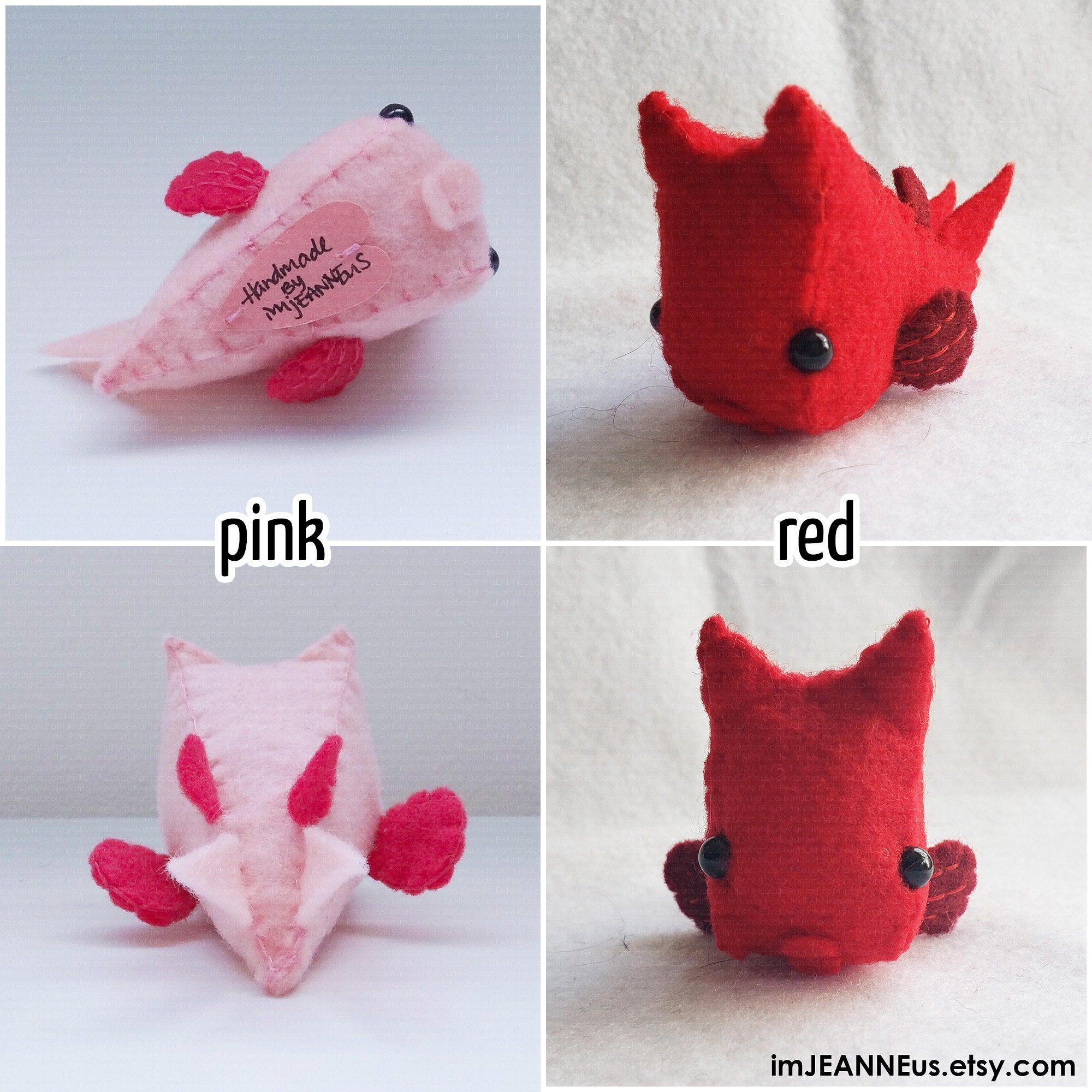This advertisement features a photo collage showcasing tiny handmade axolotls made of felt. The collage consists of four images: the two on the left present different angles of the pink axolotl, while the two on the right display various views of the red axolotl. These adorable felt creatures are designed with intricate details, including darker pink and red fins, and two black bead button eyes. Each axolotl has a tag sewn onto it, attached to a heart-shaped fabric that reads "Handmade by imgenius." Additionally, the artist's website, imgenius.etsy.com, is prominently displayed in the bottom right corner of the collage.